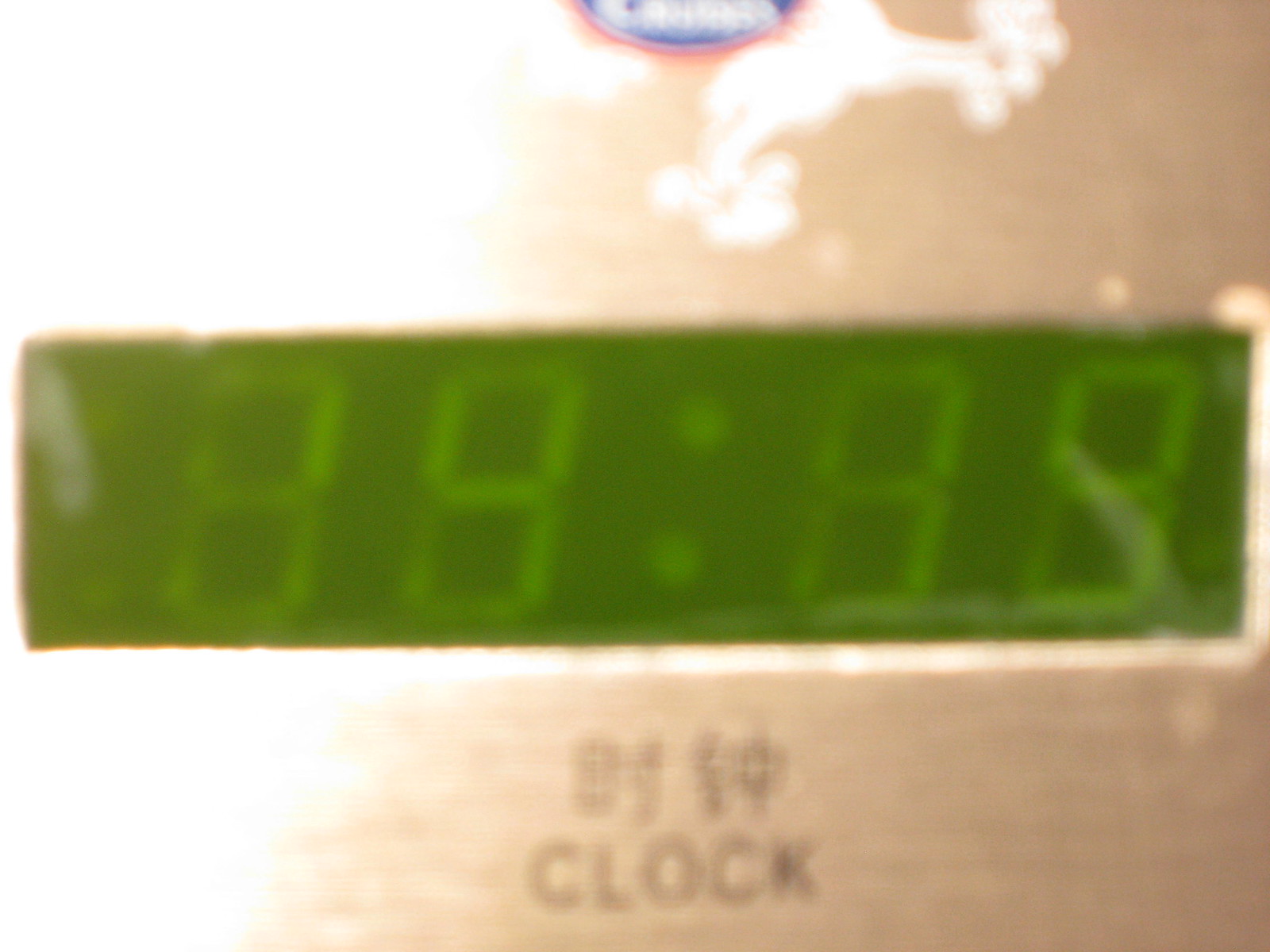A blurred close-up photograph of a digital clock is presented. The display is emitting a green hue, with the time partially discernible, possibly indicating "4:09" or a similarly structured numeral. The digits appear especially blurred, with two of them marginally bolder than the rest. Below the numbers, there is some Asian script, followed by the word "clock," seemingly engraved into the device. The extreme blurriness of the image makes the details difficult to focus on, almost inducing a sense of visual strain. At the top portion of the image, there is a cut-off blue half-circle edged with red, containing blurred white text that vaguely suggests the word "Canada." Beneath this text is an indistinct white shape that extends off to the side, adding to the overall ambiguity of the picture.